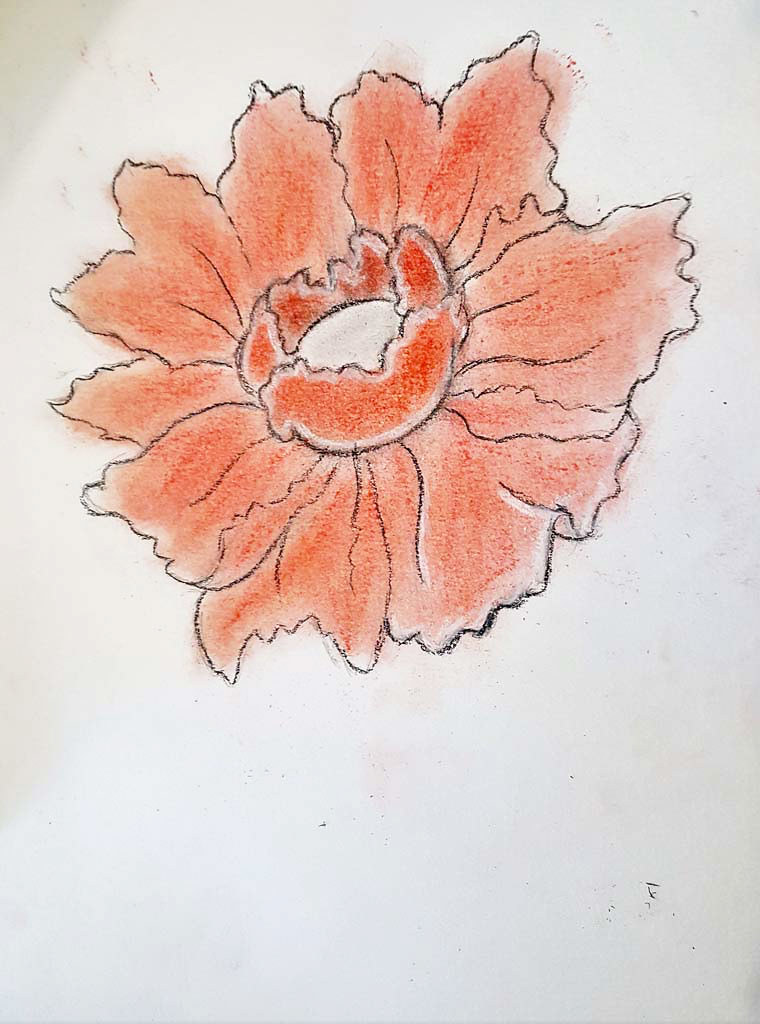This image showcases a photograph of a drawing on thick, slightly grubby white sketch paper, likely used for colored pencil drawings. The top left corner of the paper appears darker, indicating it had been previously turned over. Scattered across the paper are various blemishes and smudges, including red, blue, and pink marks, suggestive of the artist's tools touching and smearing the surface. The focal point of the drawing is a large, intricate poppy flower in the top half of the paper. The poppy, skillfully depicted in vibrant red hues, features numerous petals with rugged, ruffled edges that curve upwards, forming a cup shape. The petals are outlined in a delicate black line, possibly created with a charcoal pencil. The central section of the flower, distinguished by even redder petals, remains partially unfinished, with a stark white center. Overall, while the drawing might require further work, it already beautifully captures the delicate and detailed essence of the red bloom.